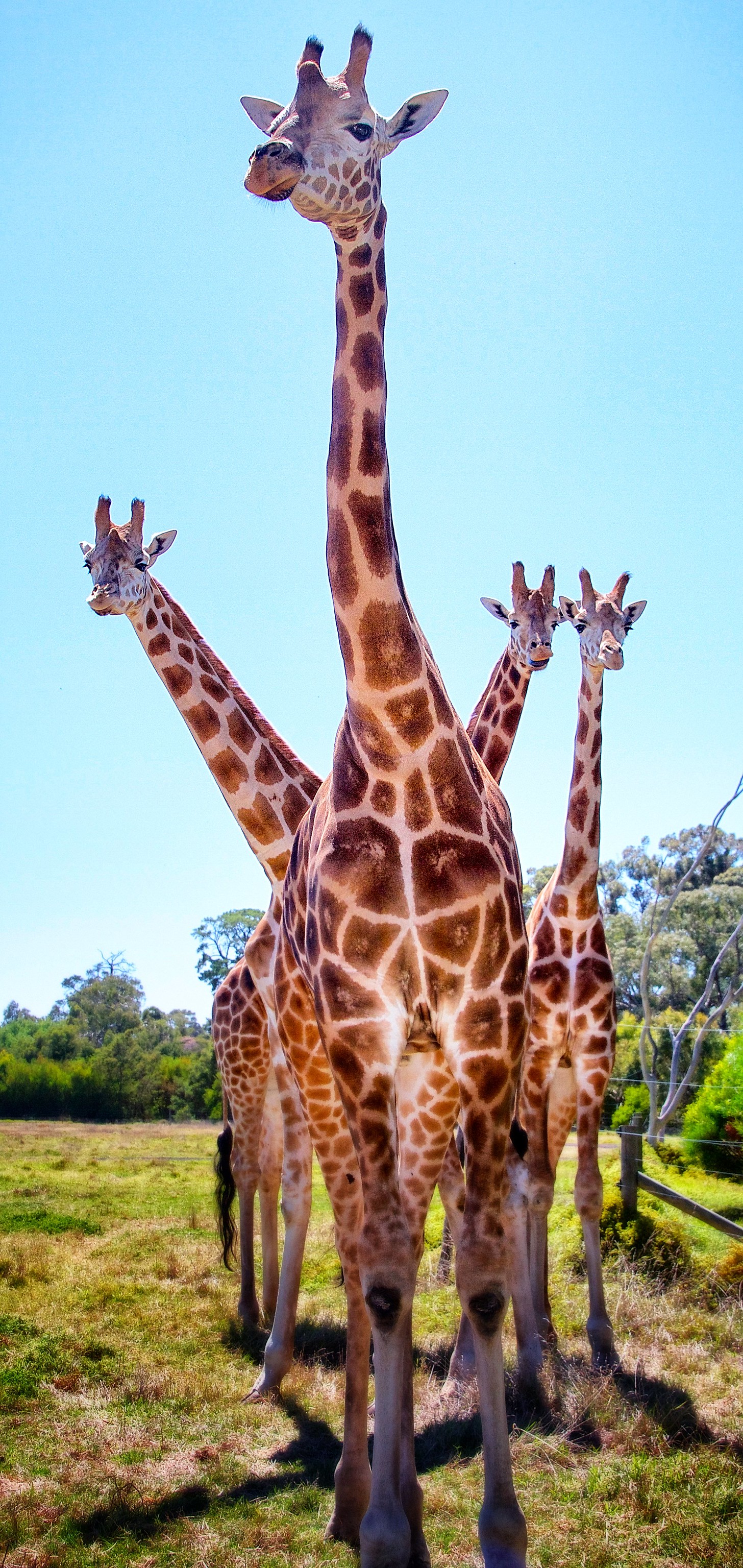In this vibrant outdoor photograph, a group of four adult giraffes stands in a large, open field. The central giraffe, closest to the viewer, nearly fills the vertical frame, its long, patterned neck extending upwards, crowned by small horns and a face that looks slightly off to the left. Its body is visible down to the ankles, and its cream-colored coat adorned with distinct orange-brown splotches shines under the high sun, casting a clear, bright light across the uneven grass below. The field exhibits patches of green, brown, and yellow, interspersed with areas of bare dirt, adding a natural texture to the scene.

Behind the central giraffe, three others align diagonally. To the left, one giraffe's neck juts upward at a 45-degree angle, prominently visible as it stretches its head towards the clear blue sky that transitions from a lighter hue near the tree line to a deeper shade above. On the right, two giraffes peek around the central figure; one reveals just its neck and head, while the other displays part of its body and its back end, distinguished by a long, black, slightly curly tail.

Flanking the scene on the right, an old fence line with three horizontal wires and what appears to be a broken fence post subtly marks the boundary. Beyond the giraffes, an assortment of tall trees and green bushes forms a lush backdrop. The trees, varying in color and height, frame the giraffes and add depth and context to the image, creating a peaceful, natural environment that might resemble a park or reserve. The overall scene is bathed in sunlight, highlighting the giraffes' distinct patterns and the rich diversity of the natural surroundings.